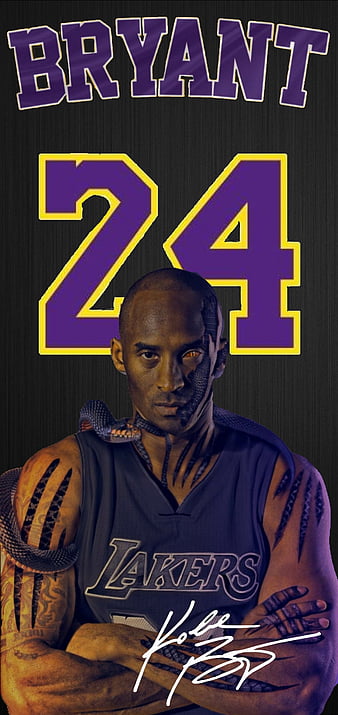The image is a detailed tribute poster dedicated to Kobe Bryant, featuring multiple elements that emphasize his legacy. The poster is tall and rectangular with a stark black background. At the top, in large capital purple letters with a white outline, it prominently displays "BRYANT," his last name. Beneath that, the number 24, one of Kobe’s iconic numbers, is written in purple with a yellow-gold outline, representing the Lakers' colors. 

The central portion of the poster features a highly detailed drawing of Kobe Bryant. In this depiction, Kobe appears to have a half-cyborg, half-snake persona. His face shows intricate scars, and he has open wounds on his arms, wrists, fingers, and neck. A black or dark purple snake, symbolizing the Black Mamba—Kobe’s nickname—is wrapped around him, possibly indicating that the markings on his body are part of his transformation into the mamba.

Kobe is shown wearing a sleeveless Lakers jersey, with tattoos visible on his muscular arms, shoulders, forearms, and fingers. His expression is serious and determined as he looks straight ahead. At the bottom right of the image, his signature appears in elegant white cursive, adding a personal touch to this professionally crafted tribute.